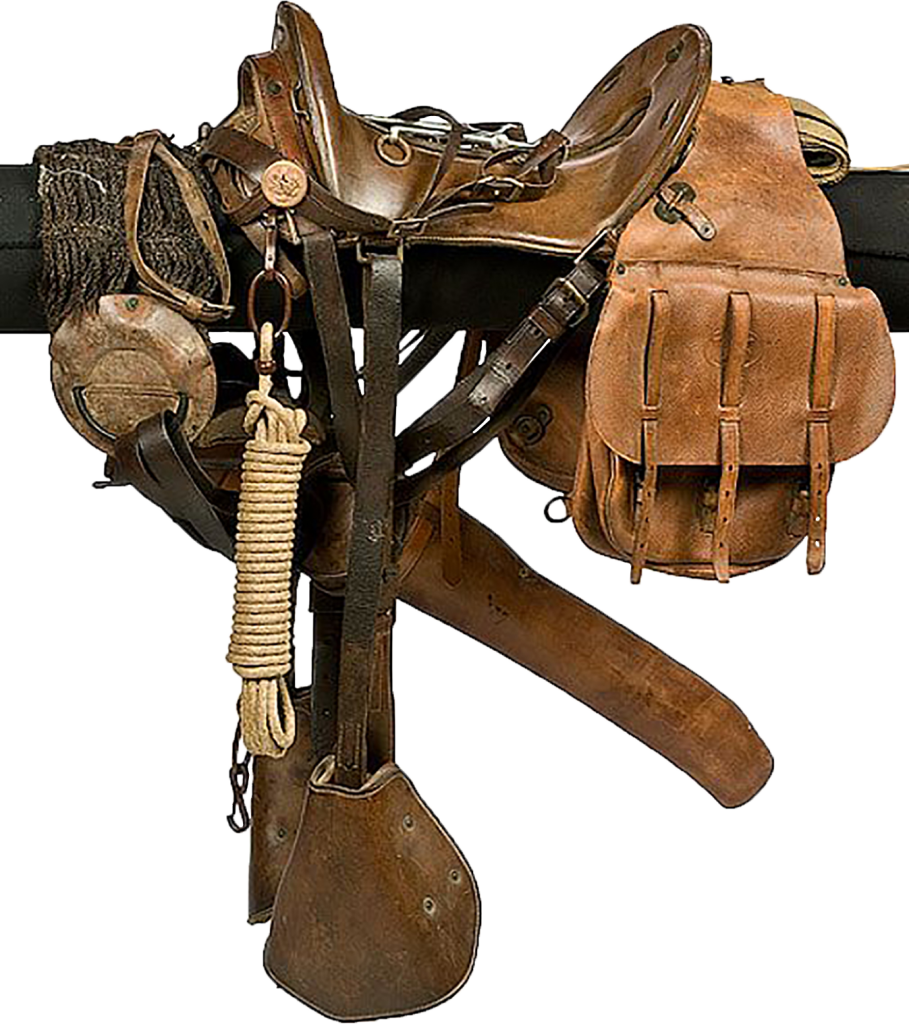A detailed photograph of a Western style horse saddle is displayed against a plain white background, seemingly floating in midair. The well-worn, dark brown leather saddle rests securely on a horizontal black wooden pole. Prominently featured are the stirrups, reins, and a variety of attached gear, all indicative of a seasoned rider's equipment. Behind the saddle sits a lighter brown, orangey leather knapsack with multiple buckles and two pouches. A tan rope, tied into a knot, hangs from a carabiner clipped to the saddle, suggesting utilitarian use. The image highlights the distressed texture of the leather and the functional, rugged design of the saddle and its accessories, capturing the essence of a country or Western riding gear setup.